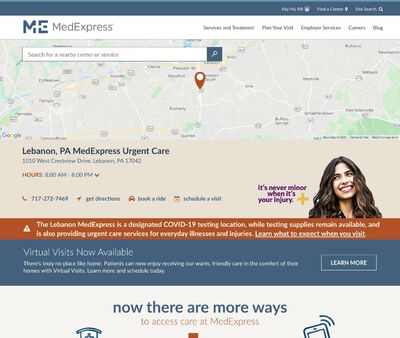Screenshot of the MedExpress Website

This image captures a screenshot from the MedExpress (ME) website. The page features a clean layout with a navigational menu next to the MedExpress logo that includes options like "Services & Treatment," "Plan Your Visit," "Exploring Services & Careers," and "Blog." At the top of the page, there’s a blue bar with additional options that are too small to read clearly.

The hero section prominently displays a Google Map inset allowing users to search for nearby MedExpress centers or specific services. One center is highlighted, indicating "Lebanon, PA MedExpress Urgent Care," along with its address and hours of operation (8 AM to 8 PM). Contact details such as the phone number are provided, and there are icons for "Get Directions," "Book a Ride," and "Schedule a Visit."

Beneath this inset, there’s a welcoming image of a Caucasian woman with brown wavy hair smiling and looking to her right. Overlaying this image is a text in purple stating, "It's never a minor injury when it's yours."

Below this section, there's a COVID-19 banner mentioning that virtual visits are now available, accompanied by a blue button prompting users to learn more.

At the very bottom of the screenshot, there’s an announcement stating, "Now there are more ways to access MedExpress," hinting at additional options like a smartphone app, although the details are cut off in the screenshot.